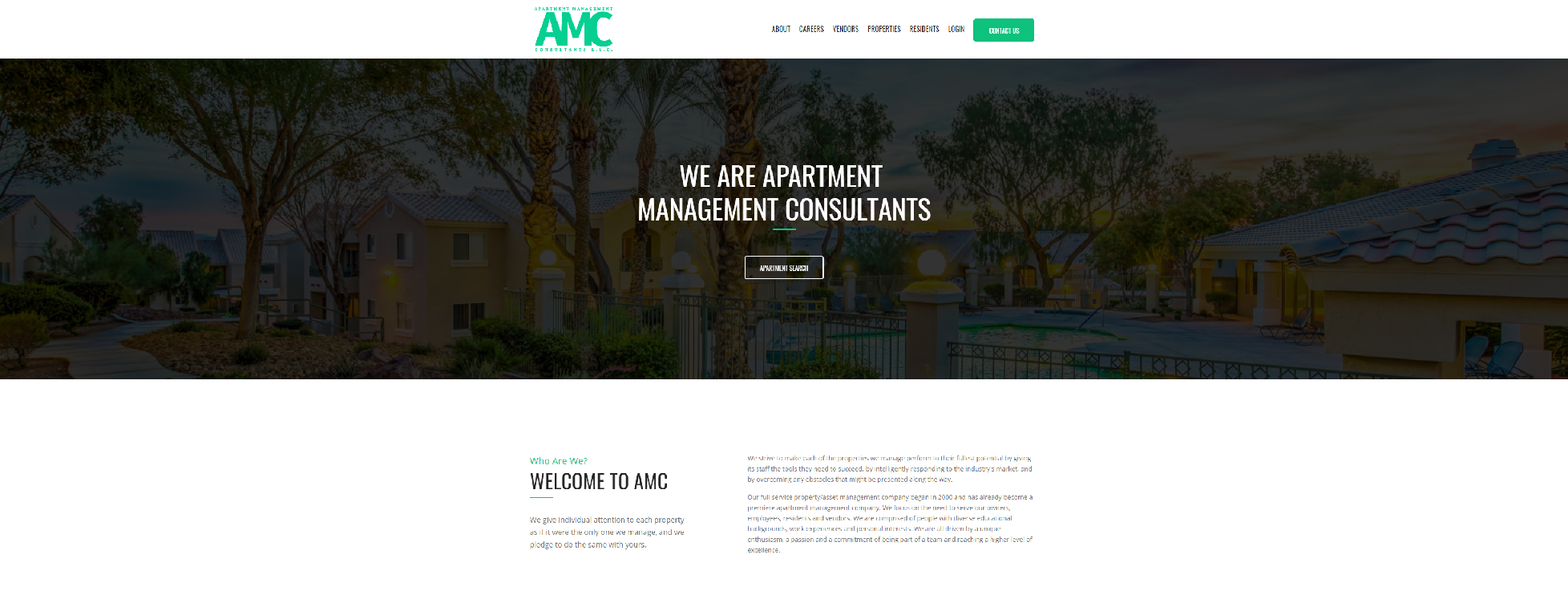This is a cropped screenshot of the Apartment Management Consultants (AMC) website, featuring a minimalist and professional design. The background is predominantly white. Positioned towards the top left center is the AMC logo, a distinct green emblem. Adjacent to the logo, slightly to the right of center, is a navigation menu with categories listed in a very small black font. Further to the right, there is a conspicuous green button. Below this header section, the top of the page includes a prominent photo background in a large rectangular frame.

Centrally overlaid on the photo is a bold text that reads, "We are Apartment Management Consultants." Beneath this tagline, a clickable box outlined in white invites interaction. Directly centered below the image, the text "Welcome to AMC" is prominently displayed in bold letters. Accompanying this welcome message is a brief description of the company. The remaining portion of the screenshot is cropped, only providing a glimpse into the layout of the desktop version of the website. The entire page appears minimized, rendering the text very small and difficult to read, suggesting that the screenshot was taken on a desktop in a wide format rather than a mobile landscape view.